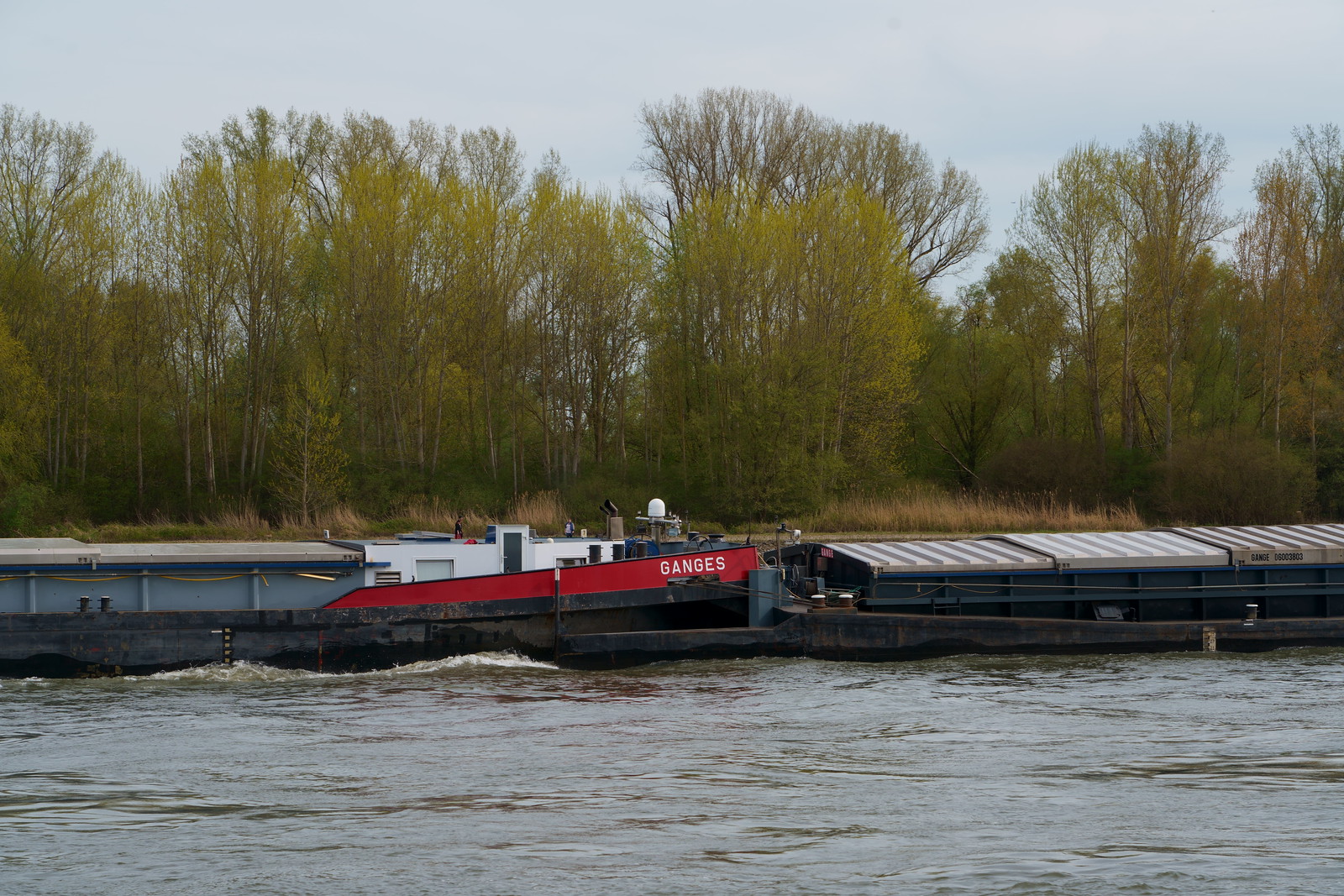Overlooking a murky brown river with noticeable currents, this photo captures a scene on a cloudy, hazy day marked by a gray sky. The riverbank is lined with buildings, starting with a prominent blue warehouse on the right side, which features a gray, corrugated metal roof extending from the center to the edge. Adjacent to this warehouse is a sequence of structures: a flat-roofed white building, a smaller white building, a small grey building, and a light blue building with a matching grey roof. Dominating the center of the composition, a large red metal frame stands tall, emblazoned with the word "Ganges" in white lettering. In the distance, a tree line consisting of tall, mostly barren trees with a sparse mix of yellow-brown leaves adds to the autumnal atmosphere. The grassy shore appears weedy and brownish. Up close, a gray low-rise building with an off-white roof and a black fence extends along the river's edge, giving the impression that it might be floating due to its proximity to the water. The overall scene exudes a somewhat dingy, late fall ambiance, with the structures and natural elements blending into the overcast day.